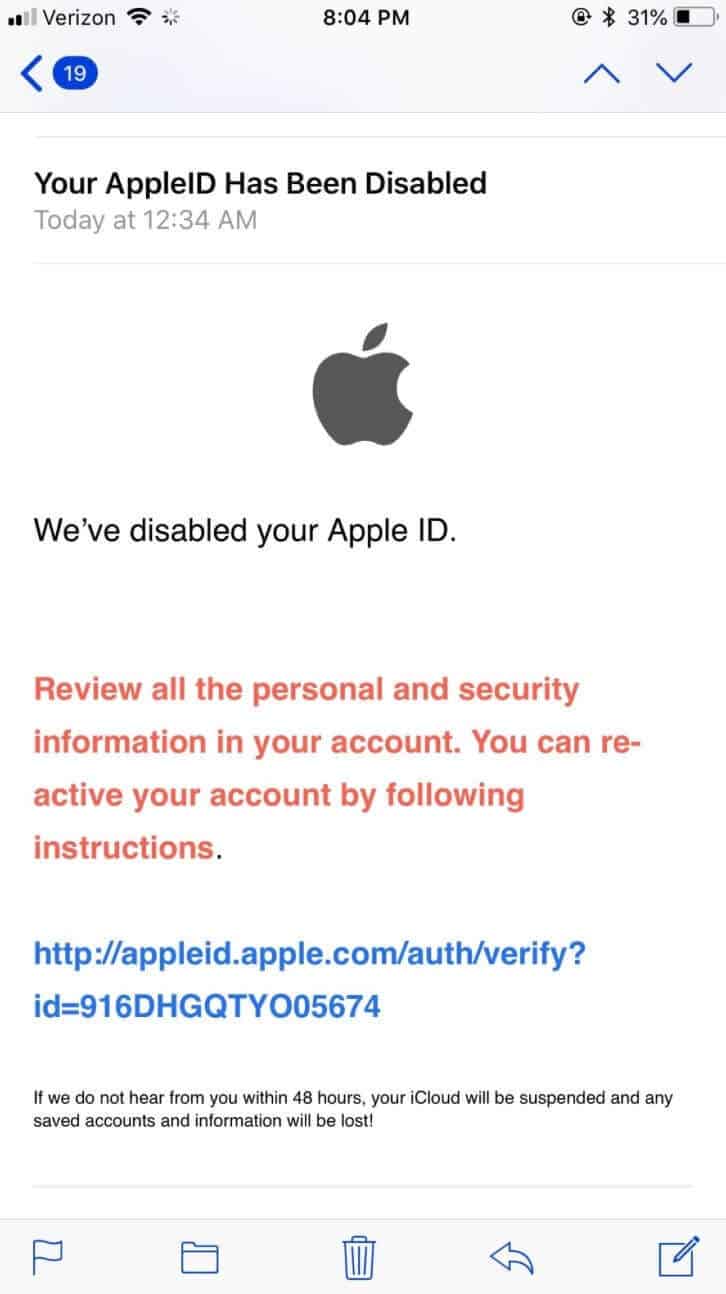A detailed screenshot of a smartphone screen appears, highlighting an email notification. The top left corner displays the Verizon network, Wi-Fi signal strength, and the time, 8:04 p.m. The battery icon shows a 31% charge. A notification indicates 19 unread messages, suggesting the content is an email.

The email is titled "Your Apple ID has been disabled," and it was received today at 12:34 a.m. Central to the image is a gray Apple logo, below which is the bold statement, "We've disabled your Apple ID." A small paragraph in red text follows, urging the recipient to review all personal and security information in their account. It mentions the possibility of reactivating the account by following provided instructions.

A blue hyperlink is visible: "http://appleid.apple.com/auth/verify" followed by an ID string consisting of numerous numbers and letters. Below this link, small black text warns that if they do not receive a response within 48 hours, the iCloud account will be suspended, and all saved accounts and information will be lost, accentuated by an exclamation point.

At the bottom of the screen, a row of icons is displayed, including flag, file, trash, reply, and write a message options.